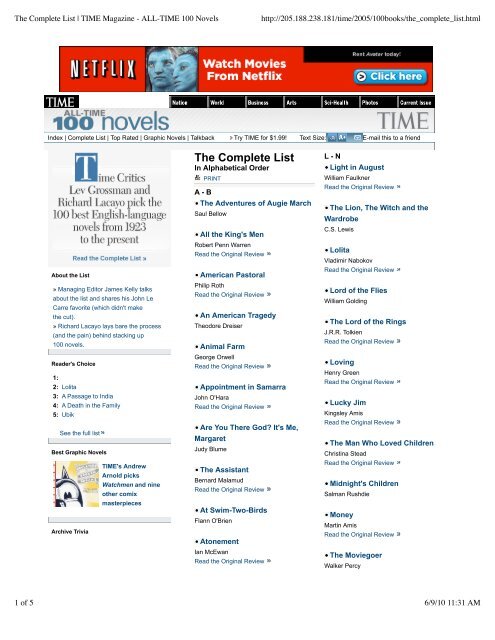The image background is primarily divided into two sections. The upper section of the background is white. On the left-hand side, there is a complete list of Time Magazine's "All-Time 100 Novels" in black text. The right-hand side features a URL—http://205188234.181-time-2005-100books-underscore-complete-underscore-list.html—though it is somewhat blurry.

In the bottom left-hand corner, there is a red rectangle with a black border. Inside this rectangle, the word "Netflix" is written in white text, outlined in black. Adjacent to this rectangle are two blue characters resembling avatars, and nearby, the text "Watch movies on Netflix" appears in white.

Below this part, there are several small black rectangles with white text inside them, but the text is unclear. The background transitions to gray toward the bottom. At the top of this section, "All Time" is written, followed by "100 Novels" in a teal color. Below that, "The Complete List" is written in black text. The list, organized in alphabetical order, includes the following titles in blue:

- A to B
- The Adventures of Augie March
- All the King's Men
- American Pastoral
- An American Tragedy
- Animal Farm
- Appointment in Samarra
- Are You There, God? It's Me, Margaret
- The Assistant
- A Death in the Family
- Atonement